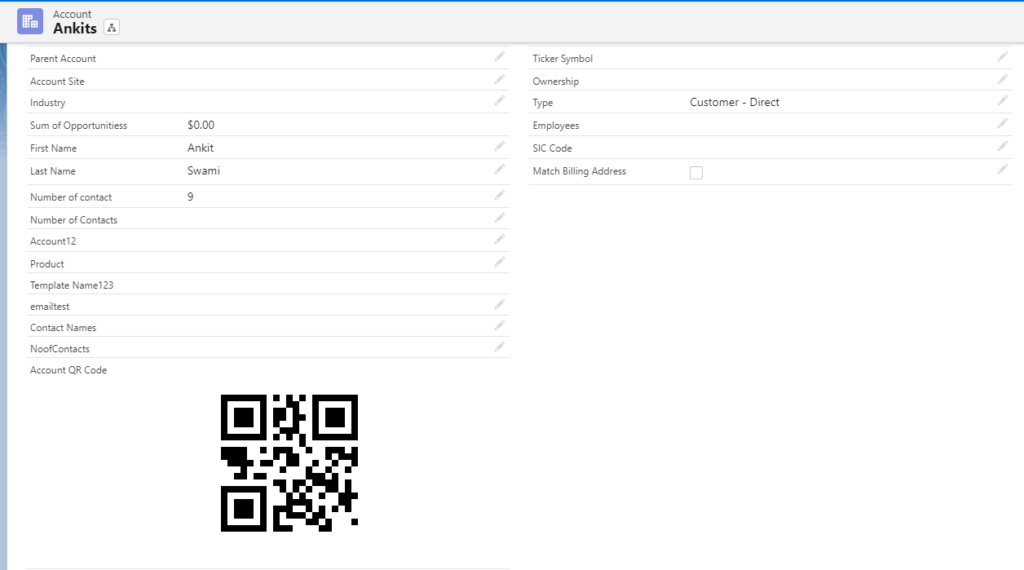The image features a clean, white background with predominantly black text positioned at the top. Below the text, there is a gray line followed by a blue line, which adds subtle separation and color to the design. A periwinkle-colored square containing a white icon stands out at the top of the image. The icon accompanies the text "Count" followed by "ANKITS" in black lettering, arranged next to a downward-pointing square.

The main section consists of a series of labels and values in black text on a white background, each accompanied by pencil symbols, likely indicating editable fields. These labels include:

- Parent Account
- Account Site
- Industry
- Sum of Operation of Opportunities: 0.0
- First Name: ANKIT
- Last Name: SWAMI
- Number of Contacts: 9
- Account: 12
- Product
- Template Name: 123
- Email Test
- Contact Names
- Number of Contacts: blank
- Account QR Code: Features a black QR code, square in shape with three prominent squares in the top-left, top-right, and bottom-left corners.

Additional details listed are:

- Ticker Symbol
- Ownership Type: Customer Direct
- Employees
- SIC Code
- Match Billing Address: followed by a blank square box

The image quality is clear, with no pixelation or graininess, making the text and details easy to read.